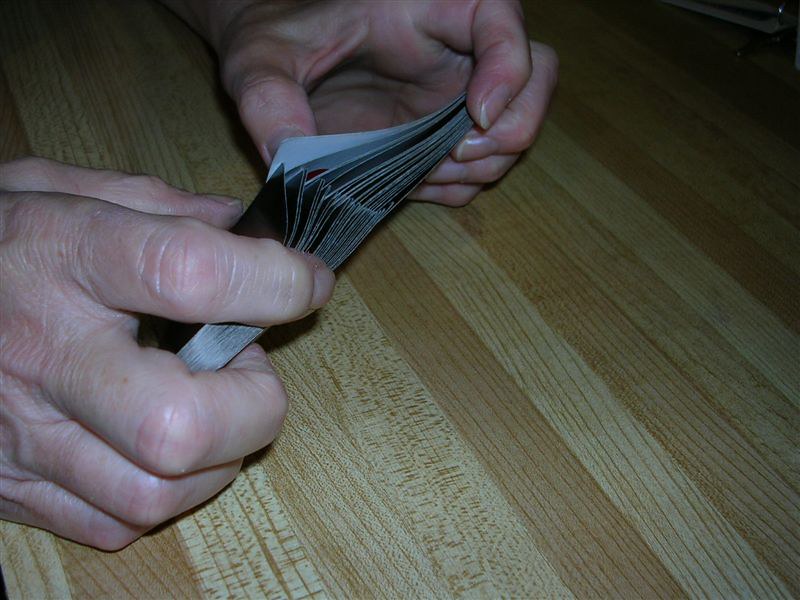The photograph captures a close-up view of a man's hands, both poised to shuffle a deck of cards. The man's skin is fair, and his fingernails are meticulously manicured and buffed to a shine. Each hand holds half of the deck, ready to combine them in a fluid shuffling motion. The table beneath his hands is made of light-stained blonde wood, adding a subtle contrast to the scene. Dim lighting casts a soft glow, highlighting the silvery sheen on the edges of the cards, which reflect the light. Although the cards' faces and backs are concealed, the visible borders shimmer elegantly. A single corner peeks through, revealing a white card face. The man's right hand grips the cards firmly, while his left hand holds them more loosely, creating a dynamic tension in this intimate moment.